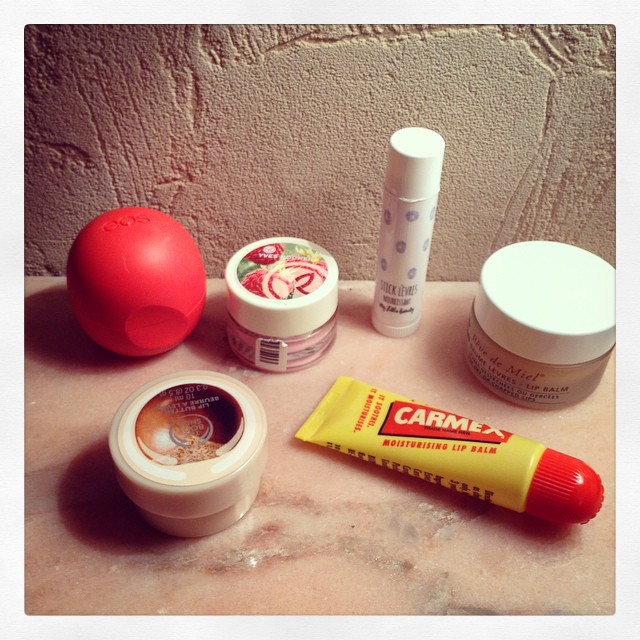This detailed color photograph, taken indoors during daytime, captures an up-close image of a pink toilet lid visibly showing areas where it has gotten wet and some rust around the metal components. The bathroom wall behind the lid is concrete, almost pink in color, adding a cohesive background tone. 

On top of the lid, there is a neatly arranged collection of personal care items. Dominating the scene is a yellow tube of Carmex with a red cap. Next to it stands a smaller, clear plastic container holding a white-lidded lip balm. Nearby is another lip balm resembling a ChapStick tube, characterized by a white body adorned with blue decorations. Then, there is a strawberry-flavored lip balm, distinguished by its iconic imagery on the lid and a caramel-flavored variant below it. Additionally, a red stress ball, appearing slightly incomplete, is positioned among the lip balms, adding an element of color contrast against the various containers on the pink lid. The overall scene gives a glimpse into a personal care arrangement in a bathroom setting.